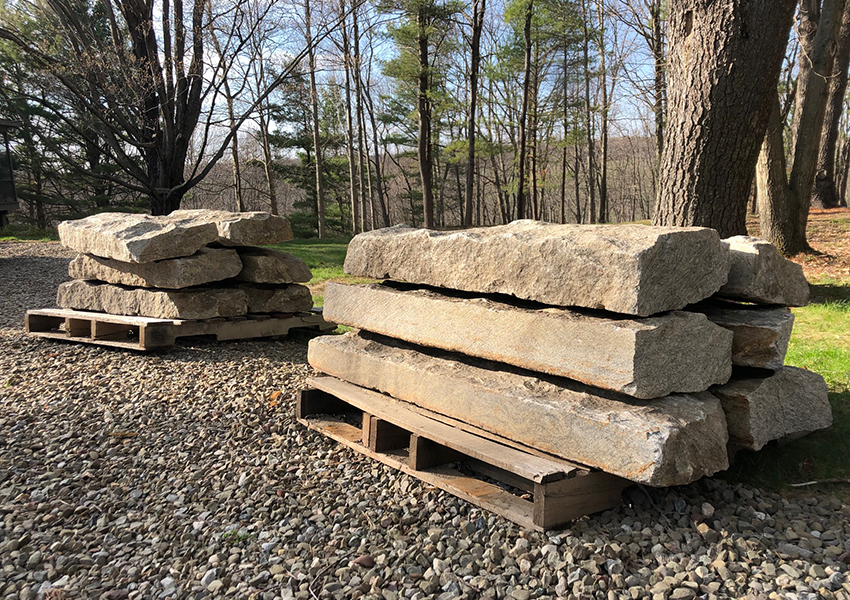This image depicts an outdoor scene with a clear rectangular orientation, with the long sides on the top and bottom. In the foreground, two wooden pallets support stacks of long, rectangular stone slabs, each pallet holding two rows of three stones, vertically piled. The slabs are roughly the size of the pallets themselves, hinting they might be intended for construction, such as building a wall or retaining structure. These pallets rest on what appears to be a gravel surface, possibly a pathway or a driveway comprising large stone gravel.

The background reveals a tranquil, natural setting with a lush forest and distant hills, suggesting a forested mountain area, possibly resembling the Appalachian Mountains. The trees are starting to regrow their leaves, indicating an early spring season. The blue sky, dotted with white clouds, peeks through the canopy, and the sunlight, perhaps from a late afternoon, bathes the scene in a warm glow. To the right, thick-trunked trees frame the image, enhancing the rustic, wooded environment.